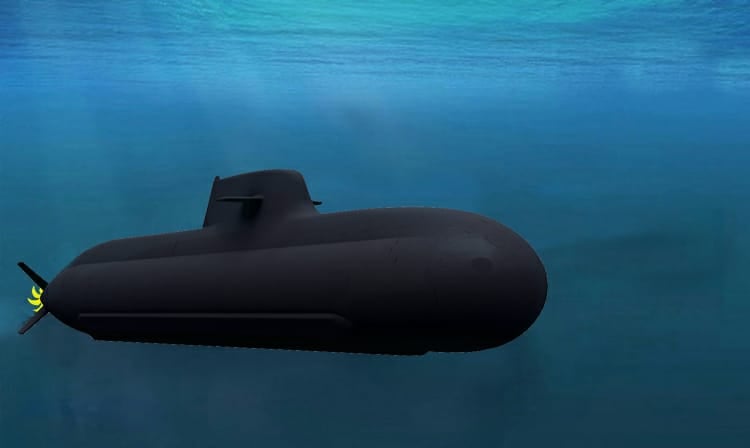The image depicts a highly detailed, 3D-rendered black submarine submerged in deep blue water with a clear gradient from dark blue at the bottom to light blue near the top, where the surface is visible and sunlight filters through. The submarine features a distinctive yellow tail with a turbine and a black triangular fin at the rear. The smooth, oval-shaped body has a rounded front and a bump on top, resembling a traditional periscope-equipped design, outlined in white with no additional ports or markings. A notable upper section, resembling a square, has two protrusions extending from it. Despite appearing stationary, there are digital artifacts around its edges, hinting at CGI origins. The contrast between the realistic water and the somewhat artificial look of the submarine, coupled with its minimalistic yet striking features, adds to the visual intrigue of the scene.